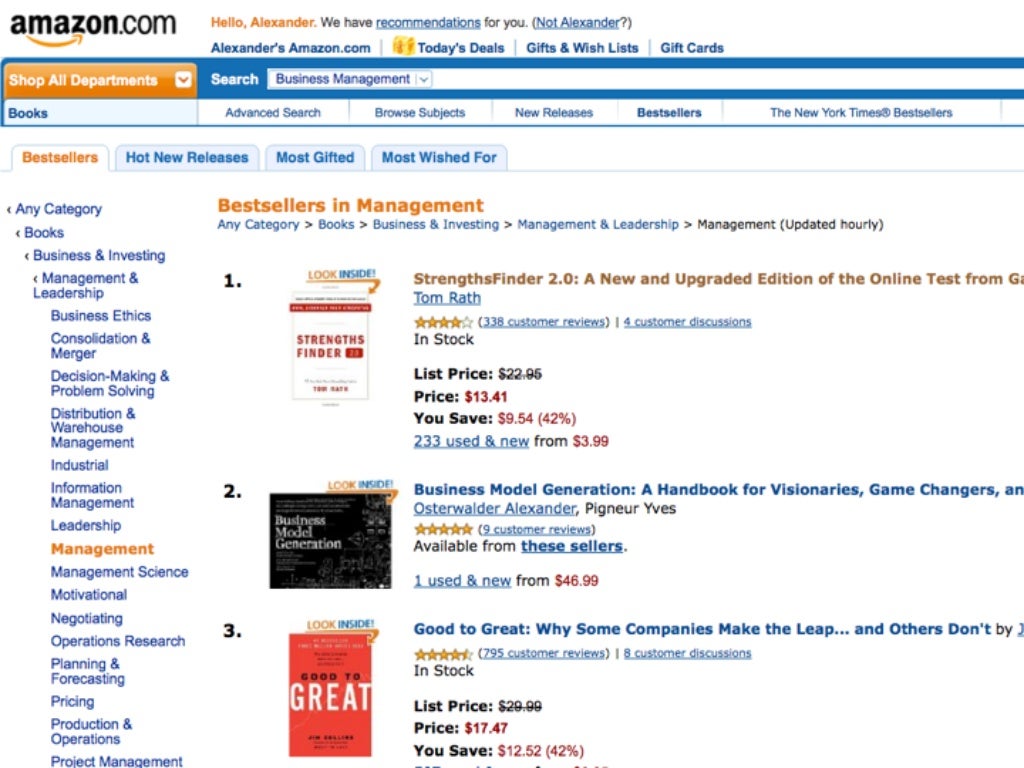This image captures a nostalgic snapshot of the Amazon website from the late 1990s or early 2000s, characterized by its simple, straightforward design. The background is plain white, and at the top, the header prominently displays the "Amazon.com" logo with the black text and the iconic orange arrow stretching from 'A' to 'Z'. Just below the logo, the site greets the user with "Hello Alexander" in orange text and suggests personalized recommendations. The navigation bar features links like "Alexander's Amazon.com," "Today's Deals," "Gifts and Wish Lists," and "Gift Cards."

Beneath this, a menu bar includes tabs for "Best Sellers," "Hot New Releases," "Most Gifted," and "Most Wished For." On the left side, a dropdown menu allows users to browse by category, currently expanded to show "Books," with "Business & Investing" and "Management & Leadership" subcategories, and "Management" highlighted in orange.

To the right of this menu, the section is titled "Best Sellers in Management," written in orange. Below this section, three books are displayed prominently:

1. "StrengthsFinder 2.0: A New and Upgraded Edition of the Online Test" by Tom Rath, with a cover image on the left.
2. "Business Model Generation: A Handbook for Visionaries, Game Changers, and Challengers," with its cover image also on the left.
3. "Good to Great: Why Some Companies Make the Leap... and Others Don't" by Jim Collins, with a cover image to its left.

These elements collectively evoke the early era of Amazon, reflecting its original focus on books before expanding into the e-commerce giant it is today.